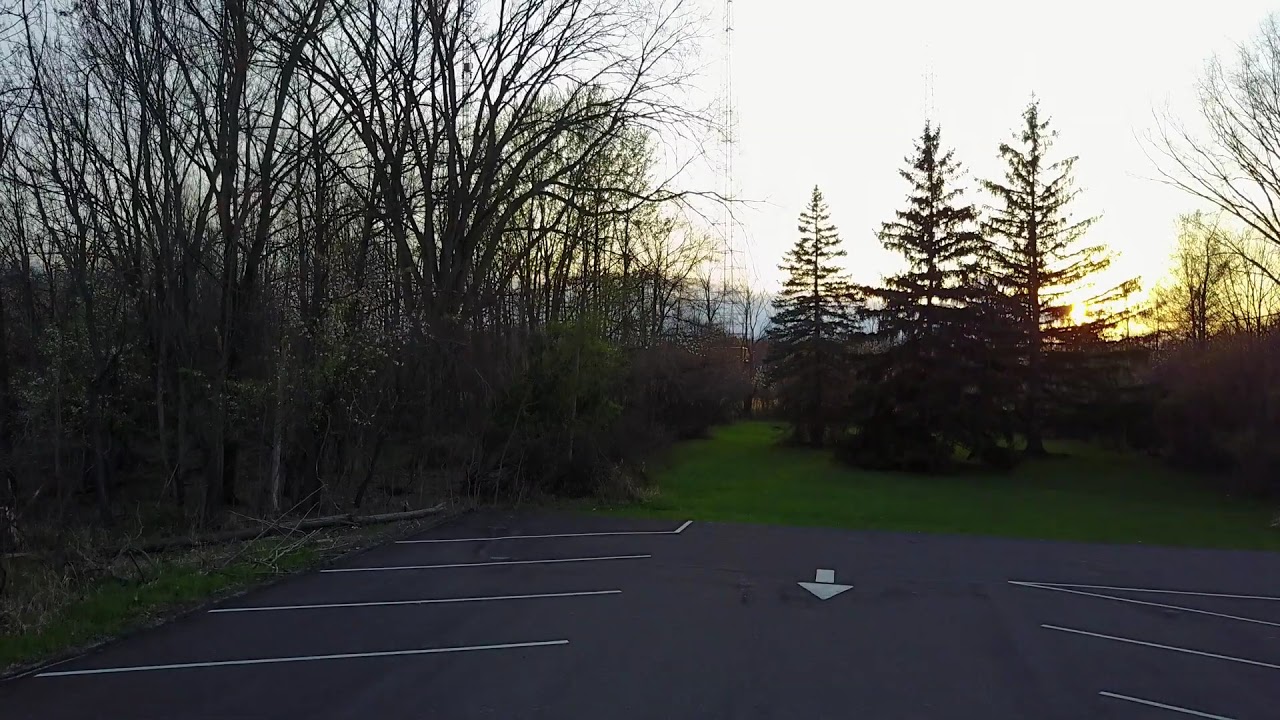This photograph, taken outdoors during the day near sunset or sunrise, captures a serene winter scene in a blacktop parking lot. The sun is very low on the horizon, casting an orange glow just above the trees and transitioning into a whitish sky. In the foreground, you see the paved parking lot featuring several white lines marking parking spaces and a white directional arrow pointing towards the bottom of the frame. Surrounding the parking lot on all sides are patches of green grass and various trees, including around four large evergreen trees with characteristic cone-like shapes. Many of the other trees are bare, indicating winter, and some fallen trees can be seen. In the background, near the left side, a thin metal structure, likely a radio or cell phone tower, rises above the tree line.